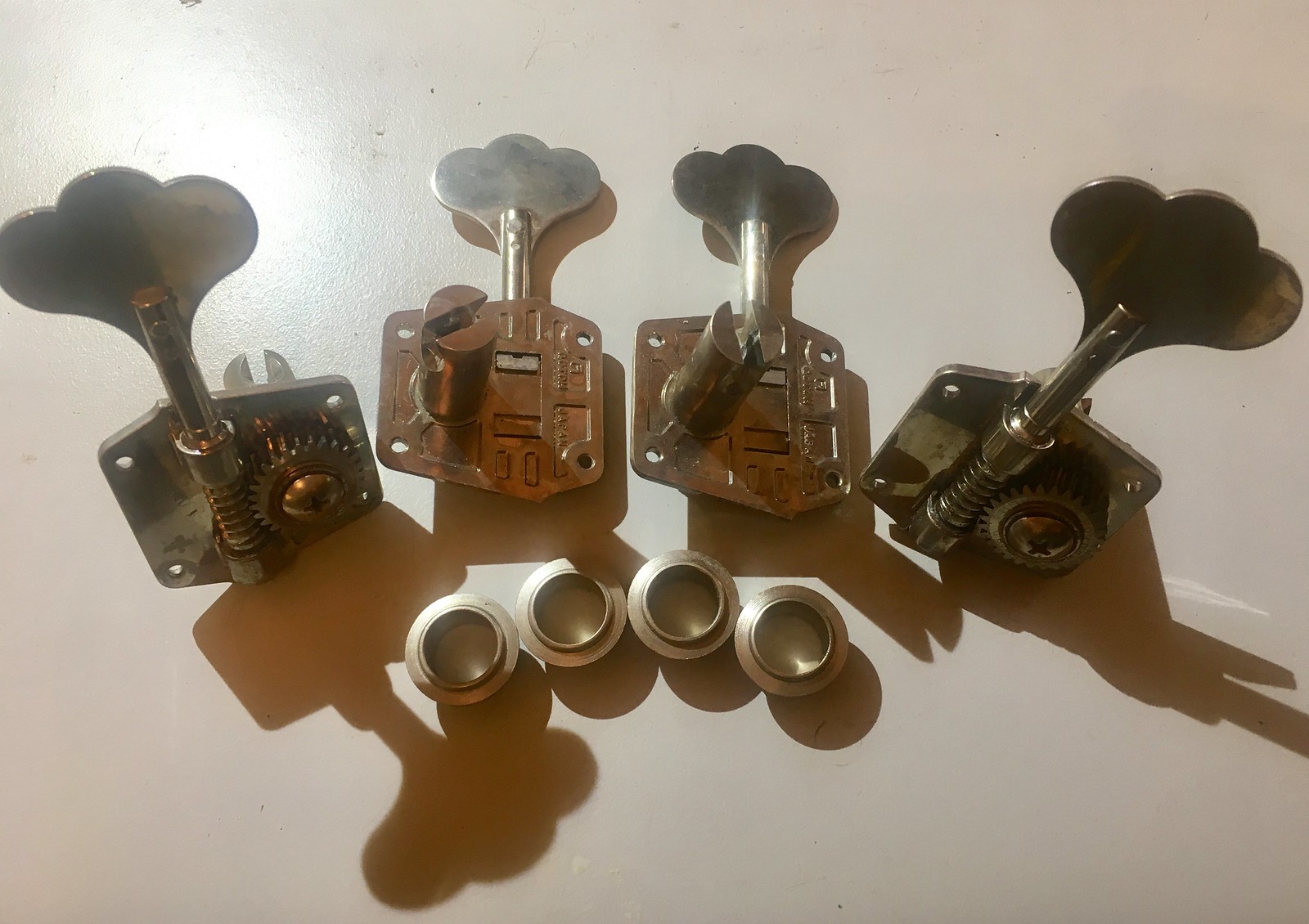The image showcases four antique-looking mechanical devices laid out on a flat white surface. These devices share a distinctive key pattern at their tops, each resembling a three-leaf clover or a mustache shape. The flat key portion leads into a cylindrical section which connects to more complex internal mechanics. Each side device reveals a visible screw-like pattern that interweaves with a gear, indicating that turning the key would, in turn, rotate the gear. 

The middle two mechanisms display an alternative view showing a cylinder with a central notch, likely turned by a hidden gear on the opposite side. Each device is mounted on a metal square base, with holes in the corners, possibly for bolts used in attachment. Below them lie four thick, dome-shaped rings, resembling the tops of doorknobs but inverted, casting strong shadows toward the bottom right, suggesting a light source from the top left. The metallic surfaces appear aged yet retain a shiny finish, hinting at their antiquity while maintaining a polished look.